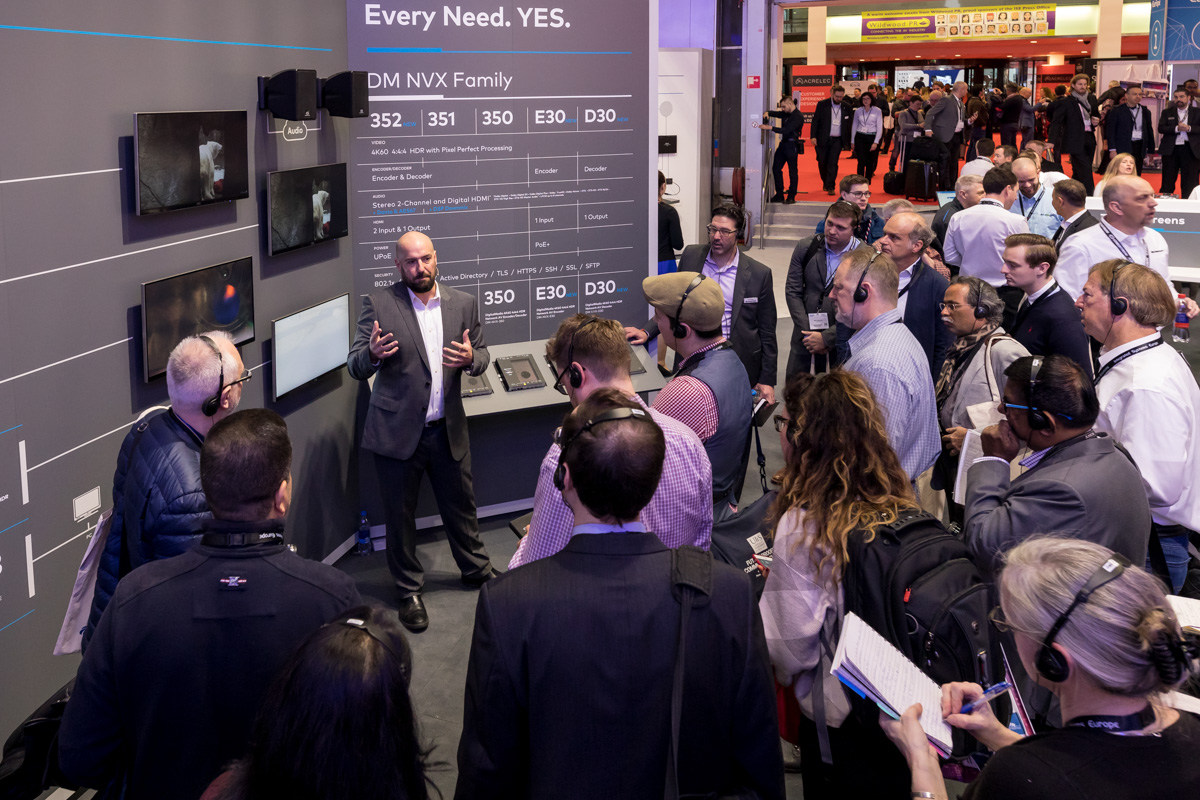A bald man with a beard and mustache, dressed in a gray suit, stands against a curved wall giving a presentation at a conference. His hands are animated as he speaks in front of a background that features multiple charts and graphs on the right and numerous TV monitors on the left. The wall also displays a sign that reads "every need, yes, DM, NVX family," along with columns labeled 352, 351, 350, E30, and D30. Surrounding him is a diverse group of engaged attendees—some with headphones and microphones, others jotting down notes or just listening attentively. These attendees sport a mix of attire, from suits to backpacks and coats. In the background, especially in the upper right corner, the bustling atmosphere of a convention hall is evident, with people walking around, some on an orange carpeted upper level. The hall is filled with a variety of colors—reds, whites, and blues—adding to the vibrant professional setting.